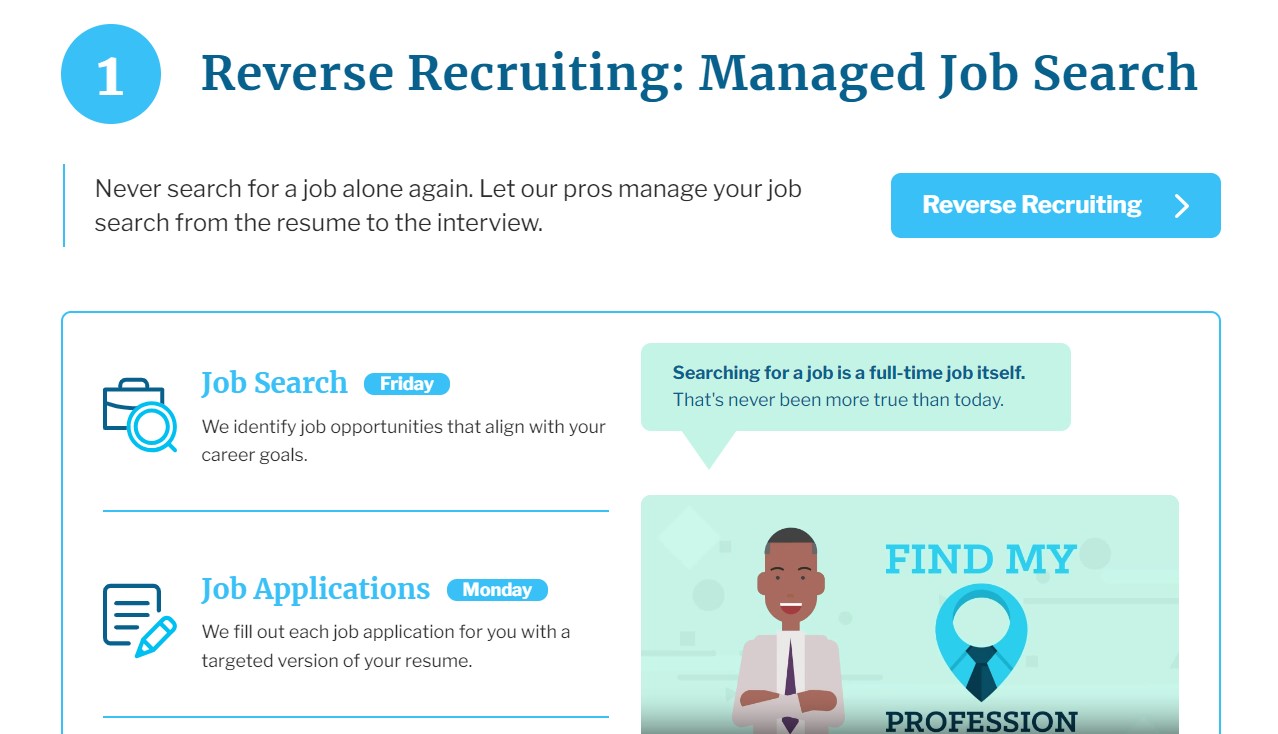This promotional page for a job search company features a clean, white background. In the upper left-hand corner, a blue circle with a white number "1" at its center stands out prominently. Adjacent to this circle, dark blue text reads, "Reverse Recruiting: Manage Job Search." Directly below this, smaller black text states, "Never search for a job alone again. Let our pros manage your job search from the resume to the interview."

To the immediate right, a blue button with white text encourages users to explore "Reverse Recruiting." Beneath this primary section, a thin blue line demarcates a different part of the page.

In the lower right-hand corner, the image of a man dressed in a tie and blazer adds a human touch. He's smiling and has his arms confidently crossed. The label near him reads, "Find My Profession." A word bubble emanates from him with the message, "Searching for a job is a full-time job itself, and that's never been more true than today."

To his left side, users are presented with two clickable options: "Job Search" and "Job Applications," making navigation intuitive and user-friendly.